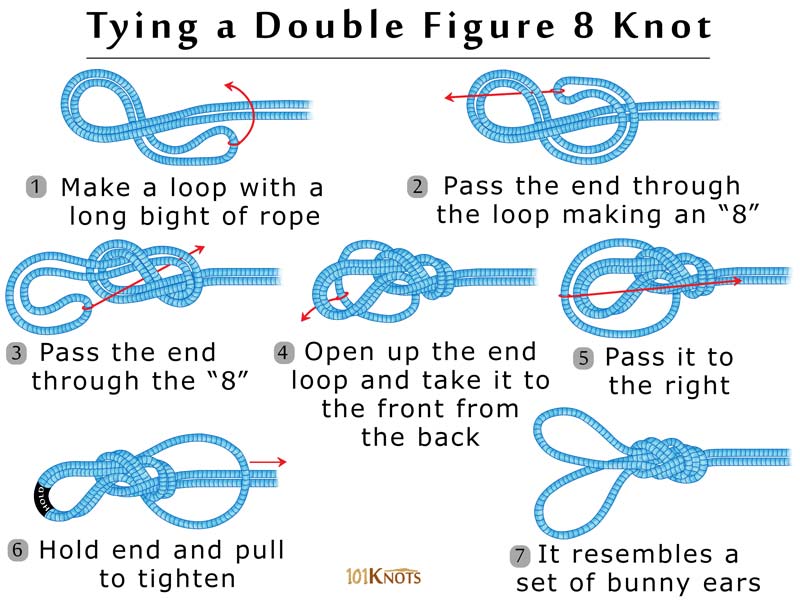The image is an instructional guide on a white background, titled "Tying a Double Figure Eight Knot" in black font at the top. Below the title, there are seven sequential images illustrating the steps to tie the knot using a blue rope. Step one instructs to "make a loop with a long bite of rope." In step two, the text reads, "pass the loop end through the loop making an eight," illustrated with a red arrow indicating the direction. Step three directs, "pass the end through the eight." Step four states, "open up the end loop and take it to the front from the back." Step five, "pass it to the right," includes an illustration with a red arrow showing the correct movement. In step six, the instruction is to "hold the end and pull to tighten." Finally, step seven notes that the knot "resembles a set of bunny ears." The bottom of the image has small golden font reading "101 Knots." The layout resembles a guide from a brochure, with images and instructions presented in a clear, step-by-step format.